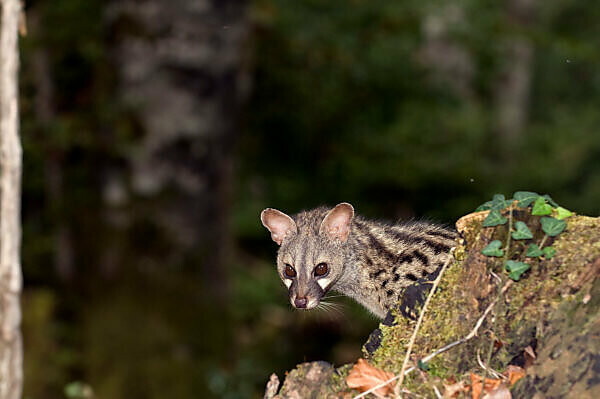The image features a small, grayish-brown mammal, likely a mongoose or similar rodent, peeking out from the top of a hole or crevice in a gray, mossy rock. Its body exhibits dark black streaks and spots, with a gray neck and face that have hints of pale brown. Prominent are its pink ears, dark brown eyes, a small nose, and whiskers. The creature is positioned in the center of the image, looking slightly downwards toward the camera. The background is heavily blurred but shows green foliage, including a tree on the left side. In the bottom middle of the photo, there's a circular watermark with an "M" on it. The lighting suggests it is either early morning or nearing nighttime.